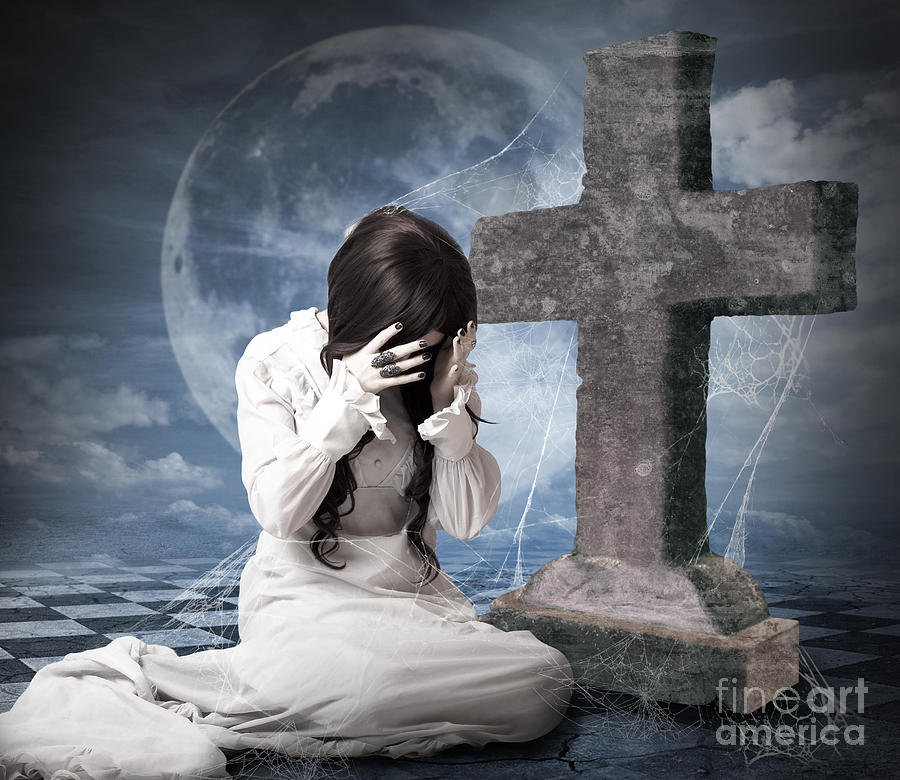This image is a detailed, emotionally-charged art piece that masterfully blends traditional photography with digital enhancements. At its center is a gothic girl with long, strikingly dark hair, dressed in a Victorian-style white dress adorned with ruffles at the wrists. Kneeling in despair, she hides her tear-streaked face in her hands, revealing black-painted nails and two dark rings on her fingers. The scene is set against a dramatic backdrop featuring a large stone cross covered in intricate cobwebs that connect to the girl, enhancing the sense of interconnected sorrow. A luminous, full blue moon hangs low in a cloudy, dark sky, while the ground beneath her is a bold black and white checkerboard pattern. In the lower right corner, the words "Fine Art America" are inscribed, marking the piece as a hauntingly beautiful example of contemporary digital art.